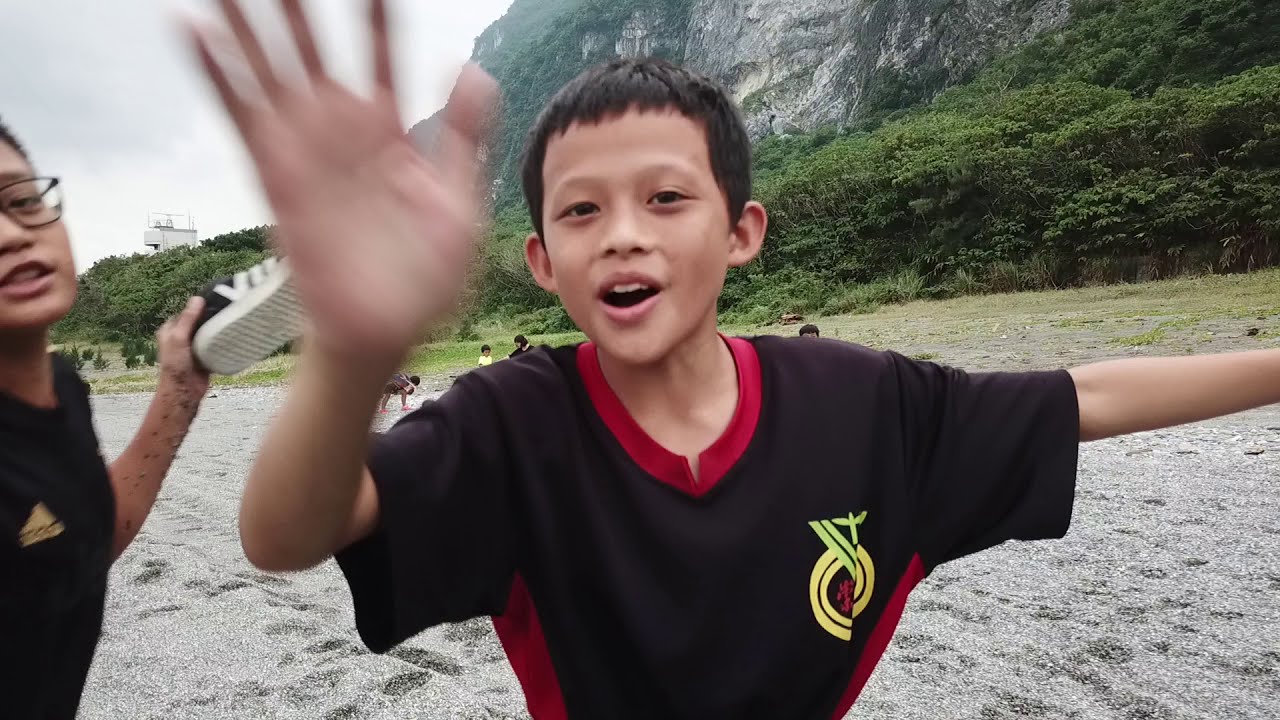The image captures two young boys, seemingly of Asian descent, enjoying a day at a beach. The boy closest to the camera has short-cropped black hair, prominent ears, and a cheerful expression as he smiles and waves his right hand. He's wearing a black shirt with a distinctive red collar and red trim, adorned with a yellow logo on the breast that appears to have some Chinese lettering. To his right, partially cut off from the frame, is another boy wearing glasses and an Adidas black t-shirt, identifiable by a yellow logo. This second boy is holding up a sneaker and has sand covering his forearm. The backdrop of the photo features a sandy beach area with people sitting nearby accompanied by a dog, alongside a tree line and a mountain under a cloudy sky, suggesting a community atmosphere.